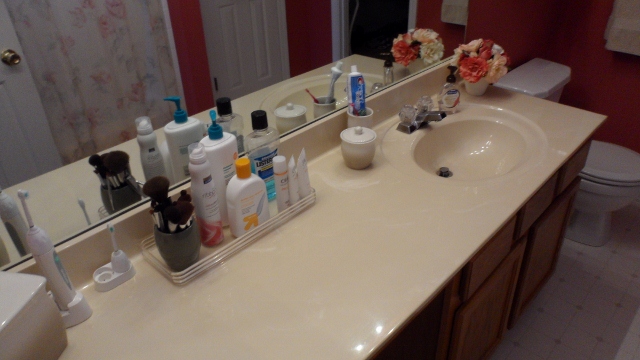In this image, we are presented with a meticulously organized bathroom space featuring a long countertop. To the right side of the counter sits a sink equipped with separate handles for hot and cold water. Adjacent to the sink, a bottle of soap is conveniently placed alongside a cup containing toothpaste and a toothbrush. Above, in the upper right-hand corner, a small pot with likely artificial flowers adds a decorative touch.

On the left-hand side of the countertop, there's a tray holding a cup filled with makeup brushes, surrounded by various skincare products, possibly lotions, and a prominently displayed bottle of blue Listerine. At the very left edge of the photo, we notice electric toothbrushes on chargers with interchangeable heads.

The far-right end of the image features a closed white toilet seat. The mirror reflects more of the bathroom, highlighting a shower curtain adorned with a floral design and a closed closet door. The overall setup suggests a well-maintained, functional, and aesthetically pleasing bathroom environment.